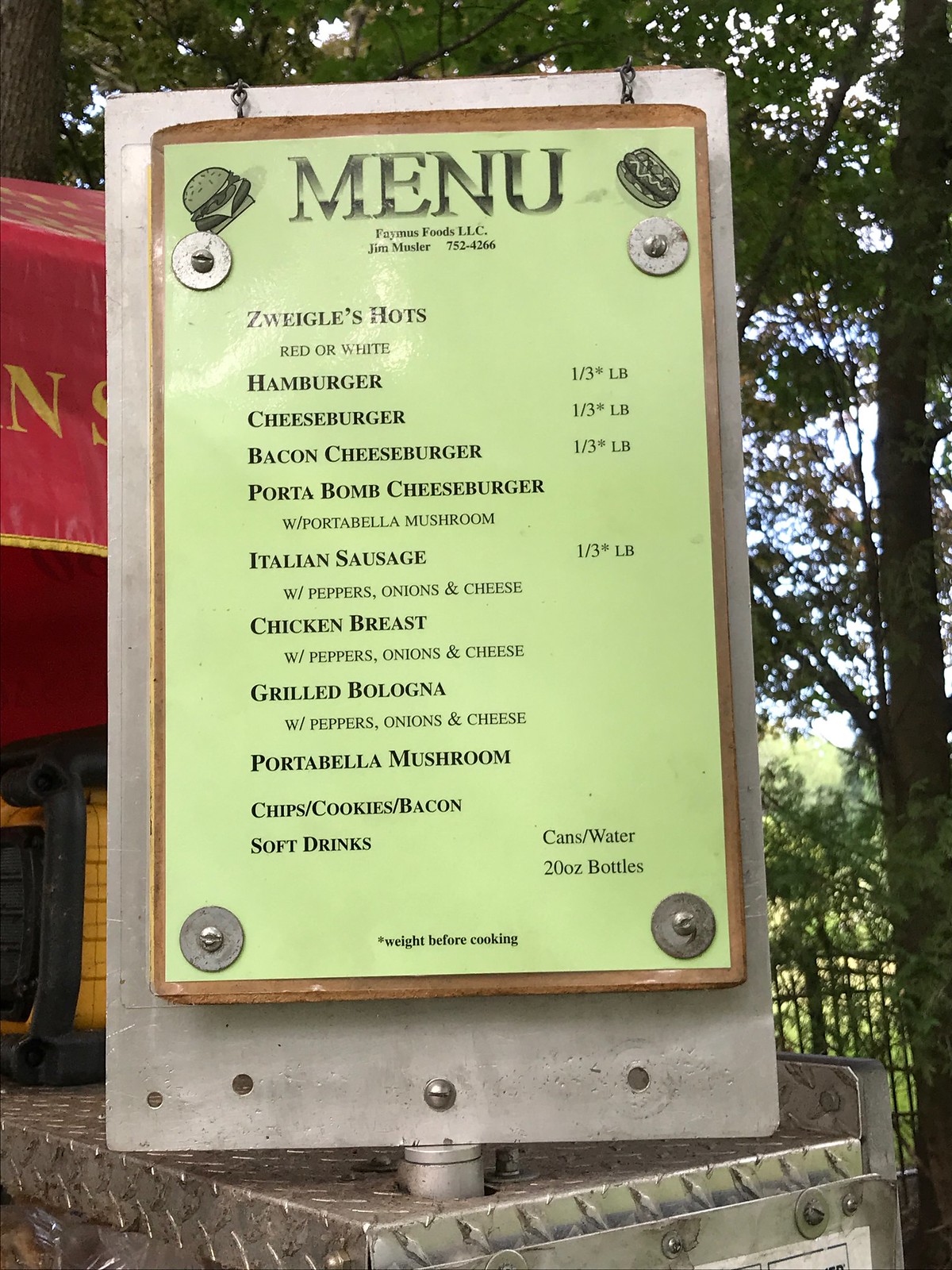This is a vibrant color photograph captured outdoors featuring a close-up view of a restaurant's menu. The menu is securely mounted on a large, oblong piece of metal, which, in turn, is attached to a metallic ledge. The menu is printed on light green paper and prominently features the word "MENU" at the top in bold letters. Although the image is slightly out of focus, several menu items are legible, including hamburger, cheeseburger, bacon cheeseburger, Italian sausage, chicken breast, grilled bologna, and portobello mushrooms. Below these items, there is a section that appears to list "soft drinks." 

In the upper left corner of the photograph, part of the restaurant building is visible, along with a red sign adorned with gold lettering. Only the letter "N" and part of the letter "S" are clear.

The background on the right side of the image offers a glimpse of a natural setting, featuring a tree trunk surrounded by a plethora of green leaves, with fragments of the sky peeking through the foliage. This harmonious blend of natural and structural elements adds depth and context to the setting of the restaurant.